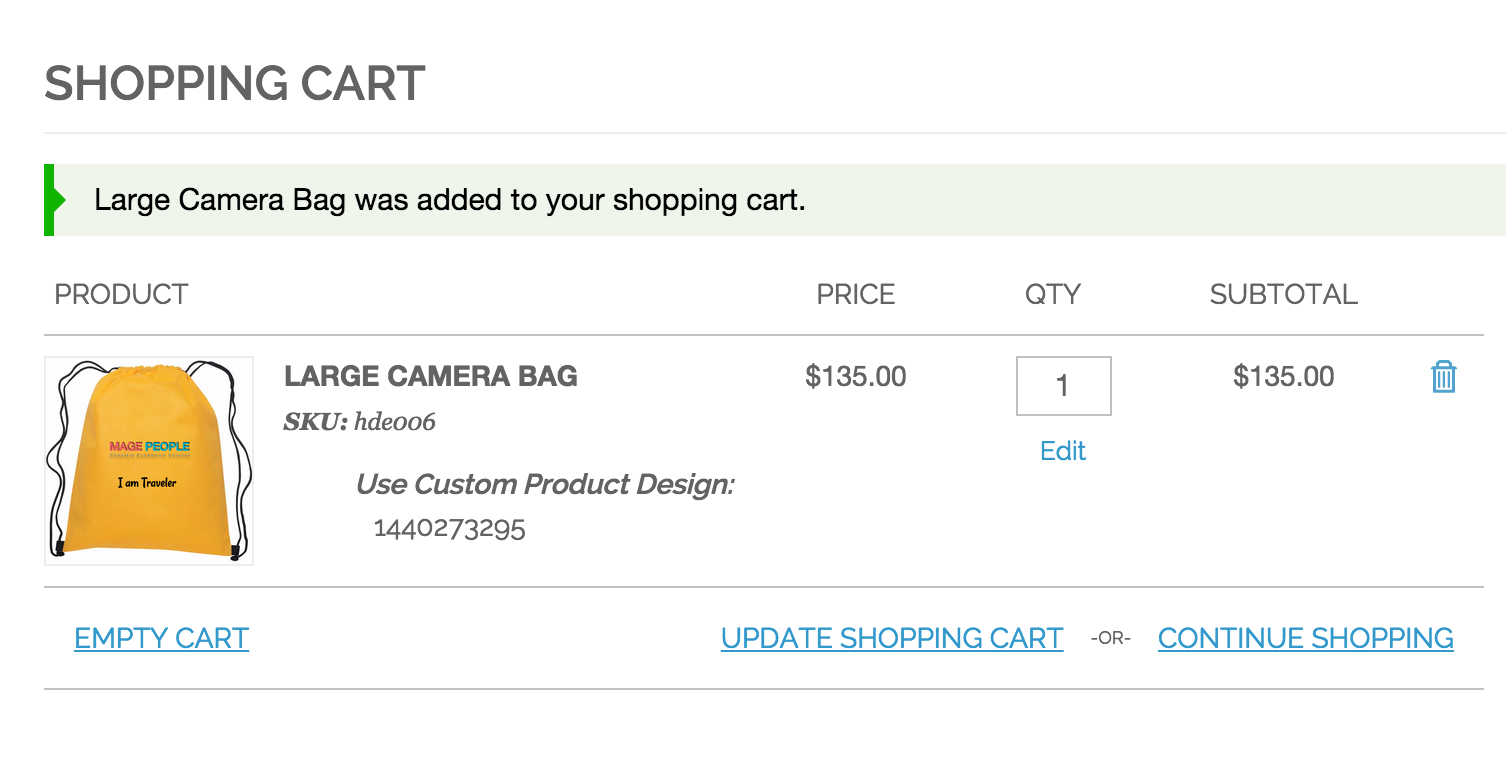This image depicts a digital shopping cart interface featuring a newly added item. At the top, bold text reads "Shopping Cart." Below this, a line divider separates the header from the main content. The top section announces in larger text that a "Large Camera Bag" has been added to the cart.

The listing is detailed as follows:
- **Product**: Large Camera Bag
- **SKU**: HDE006
- **Description**: Used custom product design 1440273295
- **Price**: $135.00
- **Quantity**: 1
- **Subtotal**: $135.00

Next to the subtotal price, there is a trash can icon, indicating a removal option for the item.

The camera bag itself is yellow, adorned with the words "MAGE" in red and "PEOPLE" in blue. Black text on the bag reads "I am traveler," and the bag's zippers and handles are also black. 

At the bottom of the screen are three options: "Empty the Cart," "Update Shopping Cart," and "Continue Shopping," enabling users to manage their shopping experience.